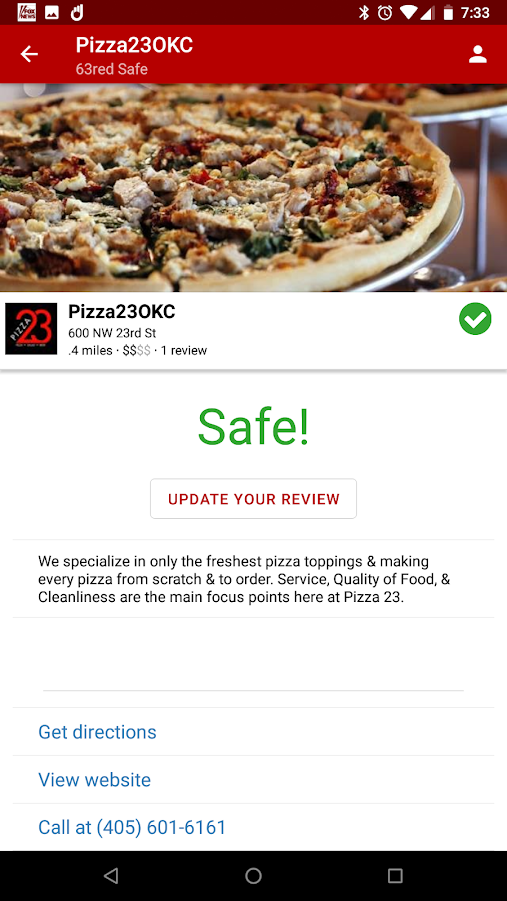The image depicts a mobile phone screen showcasing a food delivery app interface. At the very top left corner, there are icons for the app itself, a camera, and another unidentified icon. Spanning across the top header on both the left and right sides, the screen displays standard icons for Bluetooth, phone signal, Wi-Fi connectivity, cellular network strength with four bars, battery status, and the current time, which is 7:33.

Central to the screen is a profile for a restaurant named "Pizza 23 OKC." Beneath the restaurant name, the app indicates a safety status with "63 Red Safe." A prominent close-up image of a pizza on a rack follows, reinforcing the restaurant's main offering. The same safety status "Safe" is reiterated below the picture.

There is an option labeled "Update Your View," followed by a detailed description of the restaurant. Below the description, sections are available for getting directions, visiting the restaurant’s website, and making a call. The bottom of the screen features additional phone interface icons.